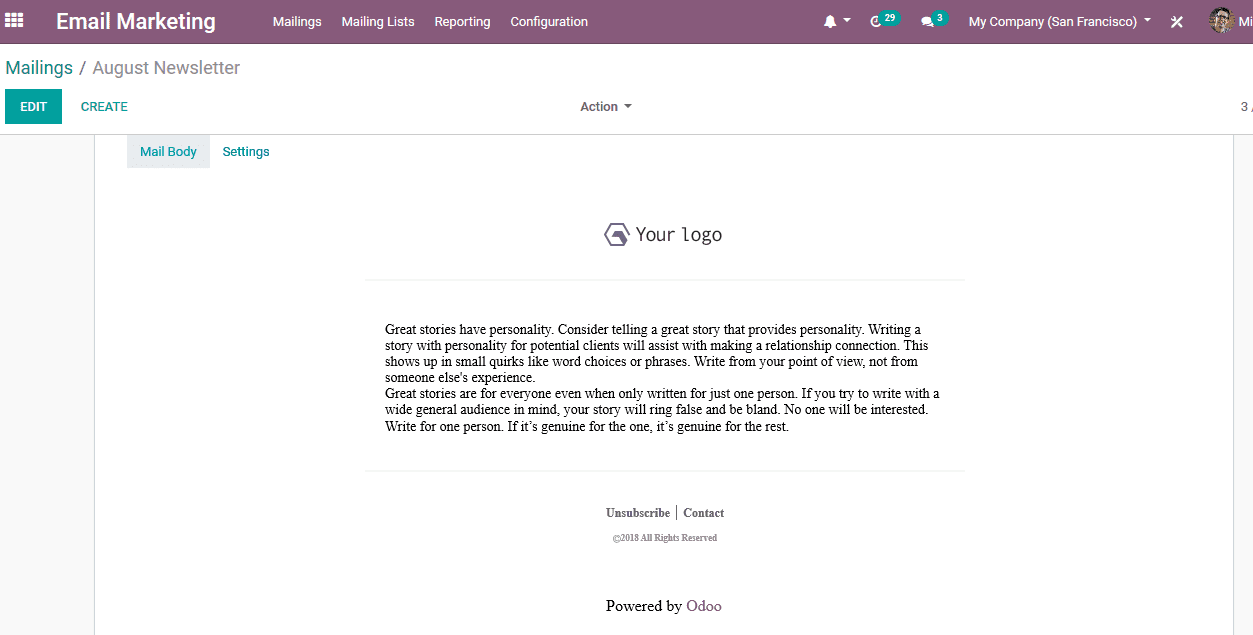**Detailed Descriptive Caption:**

The image is a screenshot of a website dedicated to generating email marketing newsletters. The page has a white background with a purple bar at the top. The bar features the title "Email Marketing" alongside four navigation tabs labeled "Mailing," "Reporting," "Configuration," and "My Company," indicating where your company is located. On the right side of the bar, there are several icons including a bell for notifications, indicating three unread notifications, a comments section with a count of three, and a timed events section showing 29 upcoming events. Additionally, there is a tool icon and a personal profile section.

Beneath the top bar, in teal font, the text reads "Mailings / August Newsletter" followed by a gray font. Below this is a toolbar with options to either "Edit" or "Create" a newsletter, with "Edit" selected and highlighted in a teal box. The newsletter in progress is displayed in the section below. 

At the top left of this section, there are two tabs: "Mail Body" and "Settings." The "Mail Body" tab is selected, marked in teal font with a gray box around it. The content area in the center of the mail body has a placeholder for inserting your logo. The main text of the mail body is a piece on the importance of storytelling in email marketing. It reads:

"Great stories have personality. Consider telling a great story that provides personality. Writing a story with personality for potential clients will assist with making a relationship connection. This shows up in small quirks like word choices or phrases. Write from your point of view, not from someone else's experience. Great stories are for everyone, even when only written for just one person. If you try to write with a wide general audience in mind, your story will ring false and be bland. No one will be interested. Write for one person. If it's genuine for the one, it's genuine for the rest."

At the bottom of the page, there are buttons for "Unsubscribe" and "Contact," as well as copyright information. The page is also marked with the text "Powered by Odoo."